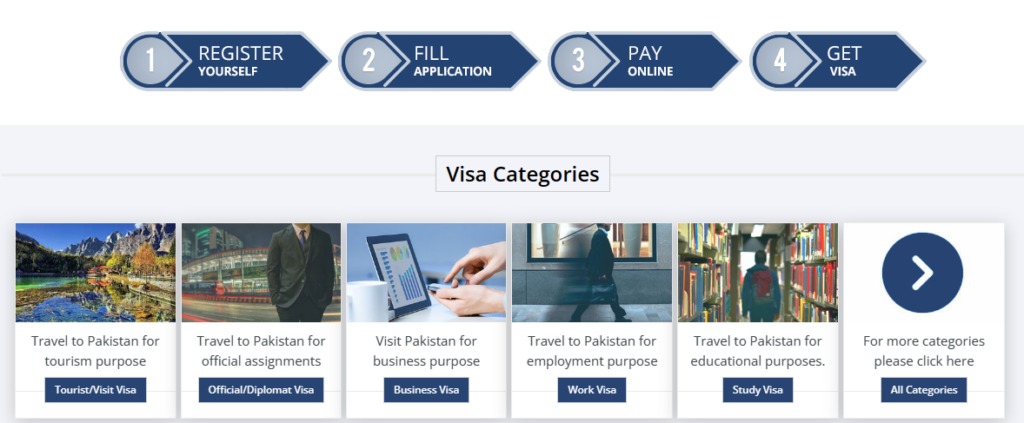The image provides detailed information about obtaining a travel visa, specifically for Pakistan. At the top, there are four numbered steps displayed within a blue strip:

1. Register Yourself
2. Fill Application
3. Pay Online
4. Get Visa

Beneath this are three distinct sections within a long, skinny horizontal gray rectangle labeled "Visa Categories." Each section features a picture and a corresponding description with a clickable button.

1. **Tourist Visit Visa:**
   - **Image:** Mountains and water
   - **Description:** "Travel to Pakistan for tourism purpose"
   - **Clickable Button:** "Tourist Visit Visa"

2. **Official/Diplomat Visa:**
   - **Image:** A building with a man in a suit (face not visible)
   - **Description:** "Travel to Pakistan for official assignments"
   - **Clickable Button:** "Official/Diplomat Visa"

3. **Business Visa:**
   - **Image:** An iPad with hands on a cell phone in the foreground
   - **Description:** "Visit Pakistan for business purpose"
   - **Clickable Button:** "Business Visa"

Each section helps users identify the type of visa they need based on their purpose of travel to Pakistan.